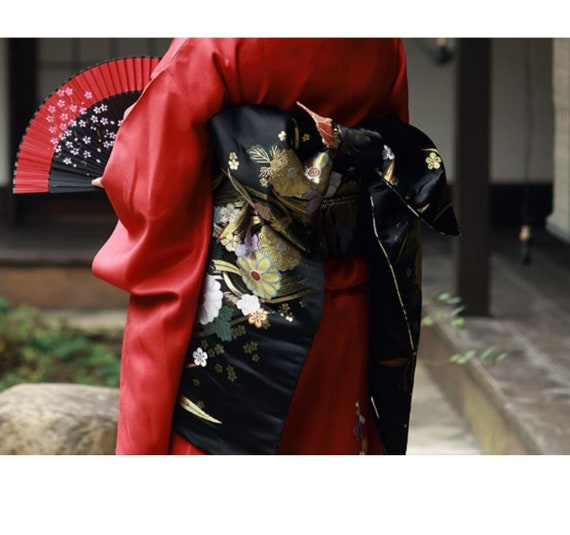In this landscape-oriented image, a woman of Asian descent is featured from the shoulders down, centered in what appears to be an indoor garden with structural elements like stone pillars and wooden posts visible in the blurry background. She is wearing a striking, bloody red kimono with a large black bow tie adorned with intricate gold, blue, and white floral designs, which extends down to cover her lower back. She holds a fan trimmed in red with a black body decorated with white stars and floral motifs, seen peeking out from behind her. Her setting includes rocks, greenery, and a sliding door to the left, contributing to the serene garden atmosphere.